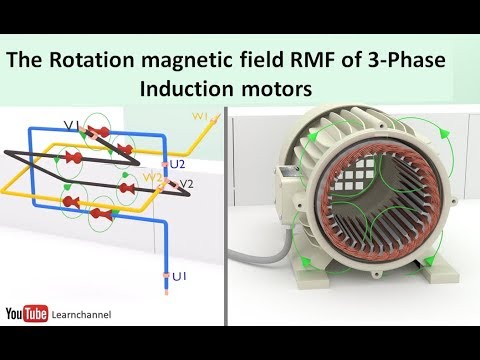The image is a detailed diagram from a YouTube video showcasing how three-phase induction motors work, sourced from the "YouTube Learn Channel". The entire image is framed with a black border on the top and bottom. Directly beneath the top black border is a light blue section featuring black text that reads: "The rotation magnetic field, RMF, of three-phase induction motors". The main content of the image is split into two sections. On the left, there is a detailed diagram with blue, yellow, and black cables labeled U1, U2, and B2 respectively, accompanied by red arrows and green circles that illustrate the electrical connections within the motor. On the right side, a photograph of a small induction motor is displayed. This motor is silver with a red inner lining visible through its open end, emphasizing the internal structure. Green arrows indicate rotational directions, and a gray power cord is visible. At the bottom left corner of the image, the text reads "YouTube Learn Channel".